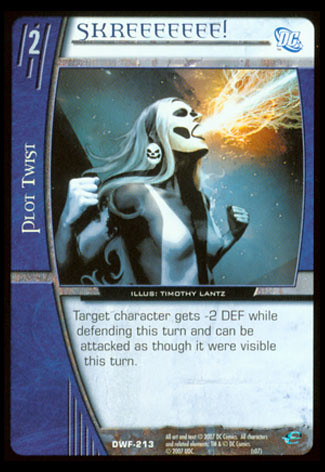The image is a computer-generated graphic of a trading card, seemingly from a game similar to Magic, featuring a female character in a dynamic superhero pose. The character, depicted in a black and white bodysuit, has long gray and green hair, a ghostly skeletal face with black eyes, and clenched fists. She is exhaling bolts of lightning and fire from her open mouth. The card's vibrant background displays a star-filled galaxy, enhancing the otherworldly atmosphere.

At the top of the card, stylized text reads "SKREEEEEE!" with an exclamation point, alongside the DC Comics logo. The right side of the card prominently features a blue element labeled "Plot Twist" with the number 2. The bottom text states: "Target character gets -2 DEF while defending this turn and can be attacked as though it were visible this turn." Additional small print includes, "ILLUS: Timothy Lance" and "DWF.213 copyright 2017," though some text remains too blurry to read clearly.